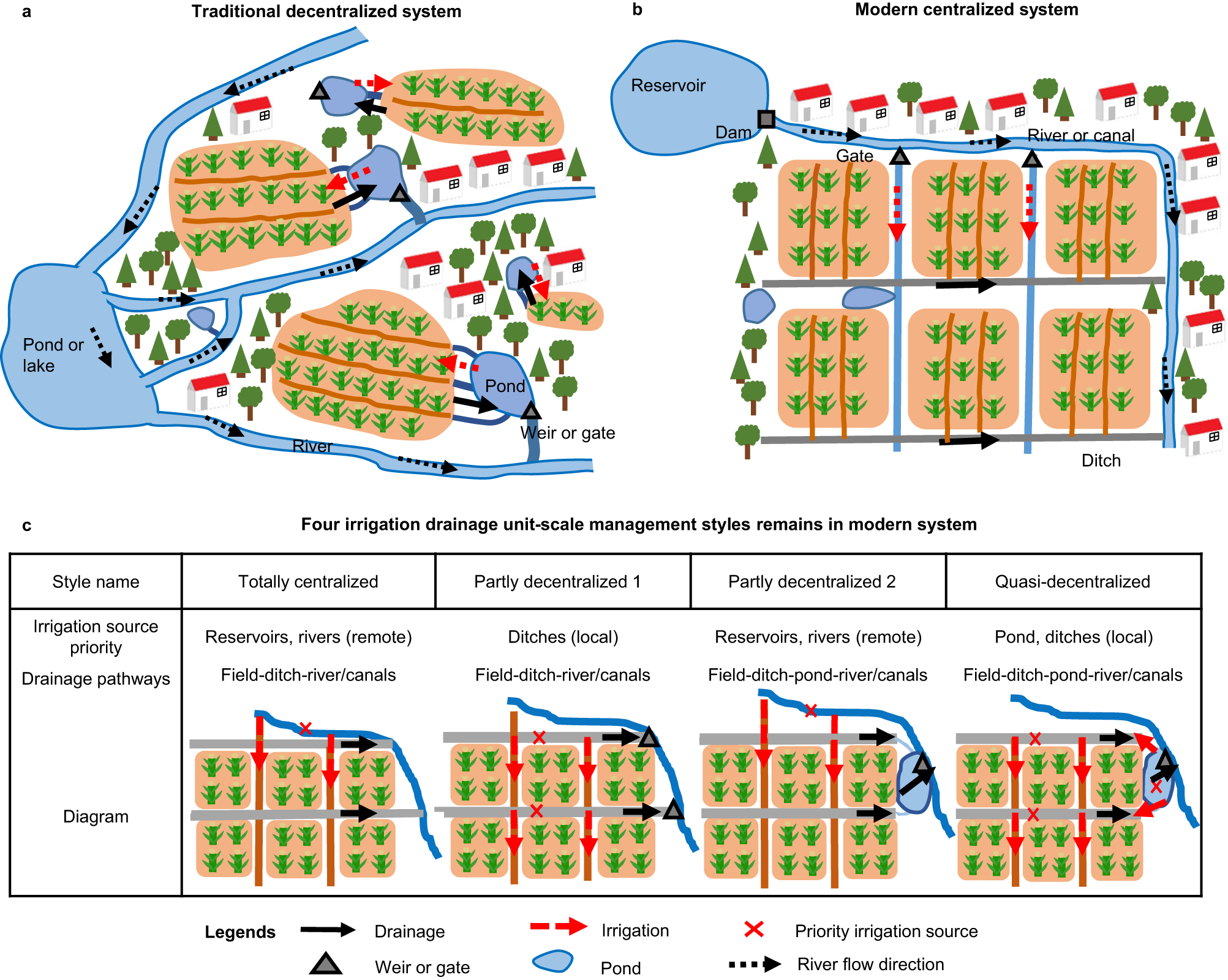The image is a detailed, multi-sectioned diagram of irrigation systems in residential areas, showcasing traditional and modern approaches to water management. At the top left (labeled A) is an illustration of a traditional decentralized system, depicting a pond from which rivers and channels distribute water to various pieces of land with homes and trees. In contrast, the top right (labeled B) features a modern centralized system. This section shows a reservoir feeding into a river or canal, which then irrigates the land in a coordinated grid pattern, also surrounded by homes and trees. At the bottom (labeled C), the diagram illustrates four types of irrigation drainage unit scale management styles used in modern systems: totally centralized, partially decentralized, partially decentralized two, and quasi-decentralized. These sub-diagrams demonstrate various irrigation patterns and water flow directions marked by different colors and symbols—green, beige, blue, red—with a detailed legend explaining the significance of black arrows for drainage, red segmented arrows for irrigation, blue circles for ponds, and more.